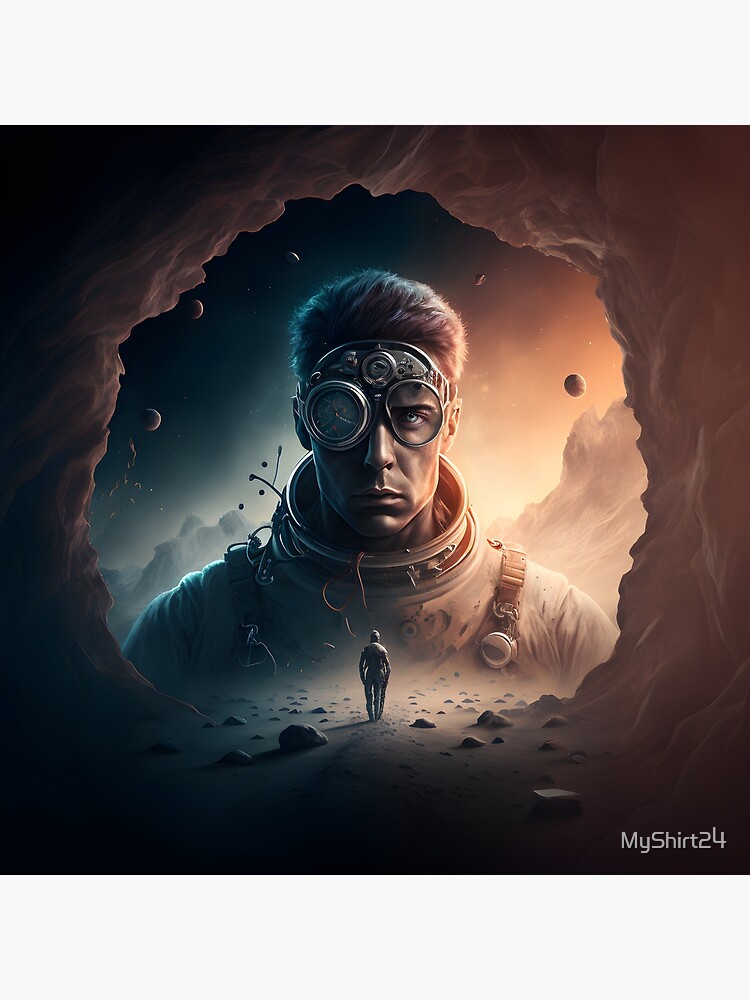This detailed dark-toned digital illustration, attributed to "MyShirt24" in white text at the bottom right corner, portrays a striking scene on an alien planet. Dominating the foreground, there is a large, futuristic astronaut-like figure depicted from the shoulders up. This young man, with short brown hair, wears advanced gear seemingly designed for rugged, rocky, and sandy environments. Notably, he has no helmet but instead sports peculiar goggles; one eye is exposed and gazing directly at the viewer, while the other is covered by a dial-like device, possibly a gauge or timepiece.

The setting appears to be inside a cave, with a large opening framing an extensive, otherworldly landscape. Through this cave entrance, a rich and vivid panorama unfolds, featuring distant mountains, clouds, and buildings. The sky of the alien planet is divided into contrasting hues—one side red and the other a bluish-black. Additionally, the sky showcases multiple planetary systems, enhancing the scene’s futuristic and surreal ambiance.